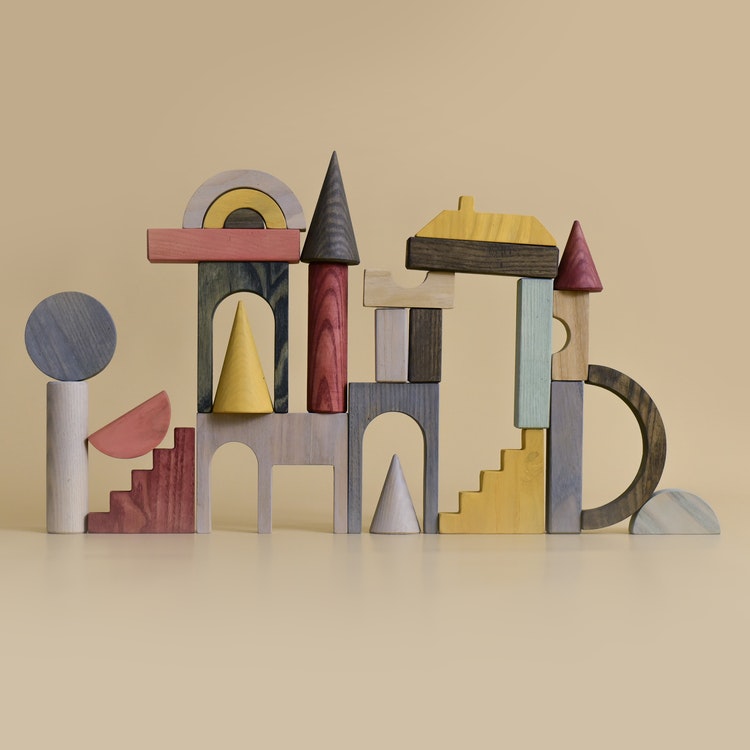The image shows an intricately crafted wooden structure positioned indoors against a beige wall and floor, resembling a castle front or stone building. Various wooden blocks of different shapes, sizes, and vibrant colors are used to form this artistic creation. Toward the left, a gray cylinder supports a dark blue sphere, while to its right, a half pink sphere is positioned alongside a gray doorway featuring two archways. Above the doorway sits a yellow conical object framed by a black archway. The right side includes a red rectangle near a maroon cylinder topped with a black triangle. The structure also includes two sets of stairs: a dark maroon stained set on the left and a lighter yellow stained set on the right. Scattered throughout the scene are additional geometric shapes, such as cones in yellow, purple, and red, adding to the complexity of the design. The composition is arranged meticulously, creating a visually captivating and detailed formation that exudes an almost fort-like appearance.